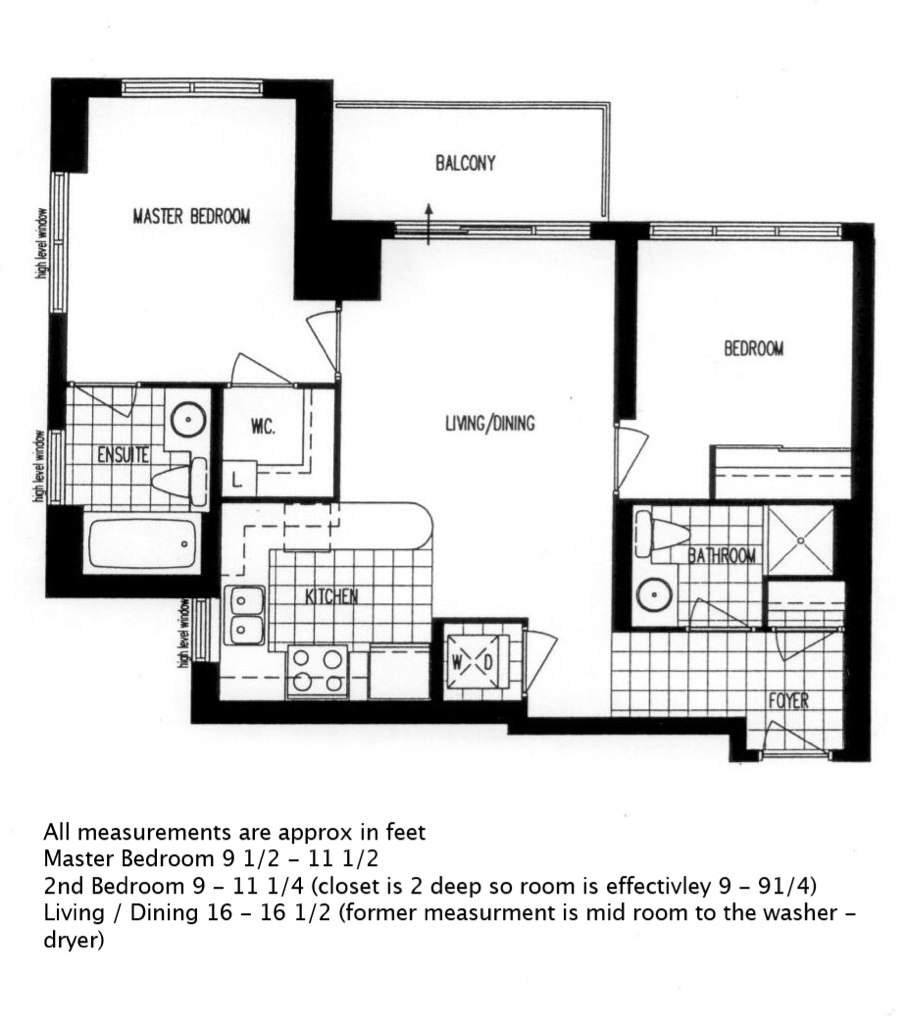The image displays a detailed black and white floor plan of a home. Each area is meticulously labeled and organized in a clockwise fashion, starting from the upper left corner. The layout includes the following spaces:

- **Master Bedroom**: Positioned in the upper left, measuring approximately 9.5 by 11.5 feet.
- **Balcony**: Adjacent to the Master Bedroom and accessible from the Living Room.
- **Second Bedroom**: Located next to the Balcony, with dimensions around 9 by 11.25 feet. The deep closet reduces the room's effective size to about 9 by 9.25 feet.
- **Bathroom**: Situated near the Second Bedroom, featuring small squares symbolizing tiled flooring.
- **Foyer**: Situated centrally, with similar tiling indicated by small squares.
- **Living/Dining Room**: Irregularly shaped with all straight lines, located in the center of the floor plan. It measures approximately 16 by 16.5 feet, with the former measurement extending midroom to the washer/dryer.
- **Kitchen**: Positioned near the Foyer and detailed with tiled flooring.
- **WC (Restroom)**: Another tiled area located adjacent to the Kitchen.
- **Suite Bathroom**: Positioned near the Master Bedroom, also featuring tiled flooring.

Additionally, the bottom of the floor plan includes a note: “All measurements are approximate and in feet.”